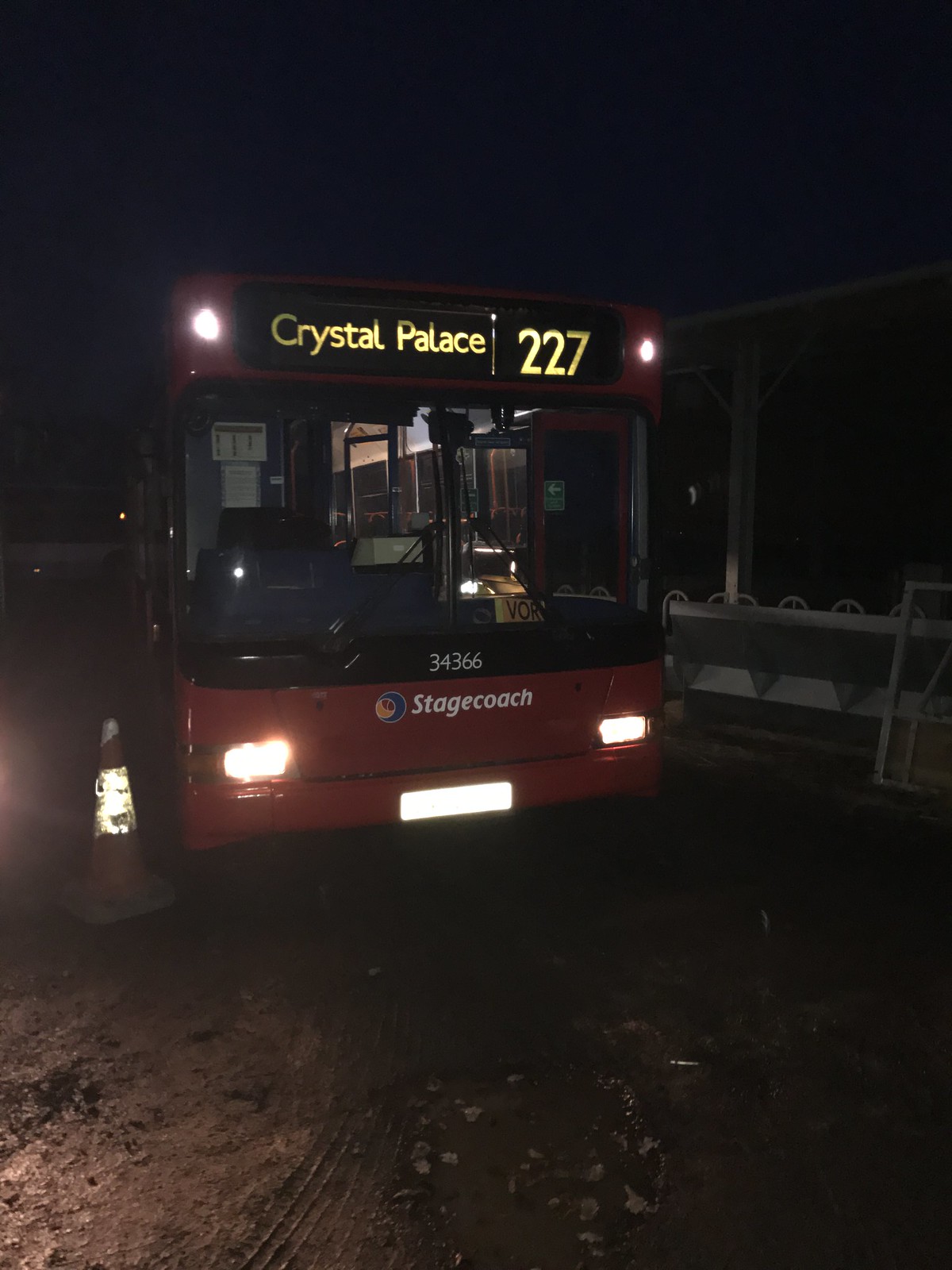In this nighttime photograph, a red Stagecoach bus numbered 34366 is parked on a dirt and rock surface. The destination display at the top of the bus reads "Crystal Palace 227" in yellow text. The bus is illuminated by its headlights, shining brightly in the dark surroundings, and additional lights are visible at both the top and bottom of the bus. An orange caution cone is positioned in the lower left corner of the image, near the front right side of the bus. The sky is pitch black, and the ground shows signs of tire tracks and scattered rocks. There is a shadowy outline of a building on the right side of the image, adding to the overall dark and quiet ambiance. The bus appears stationary, and there are no passengers visible inside.